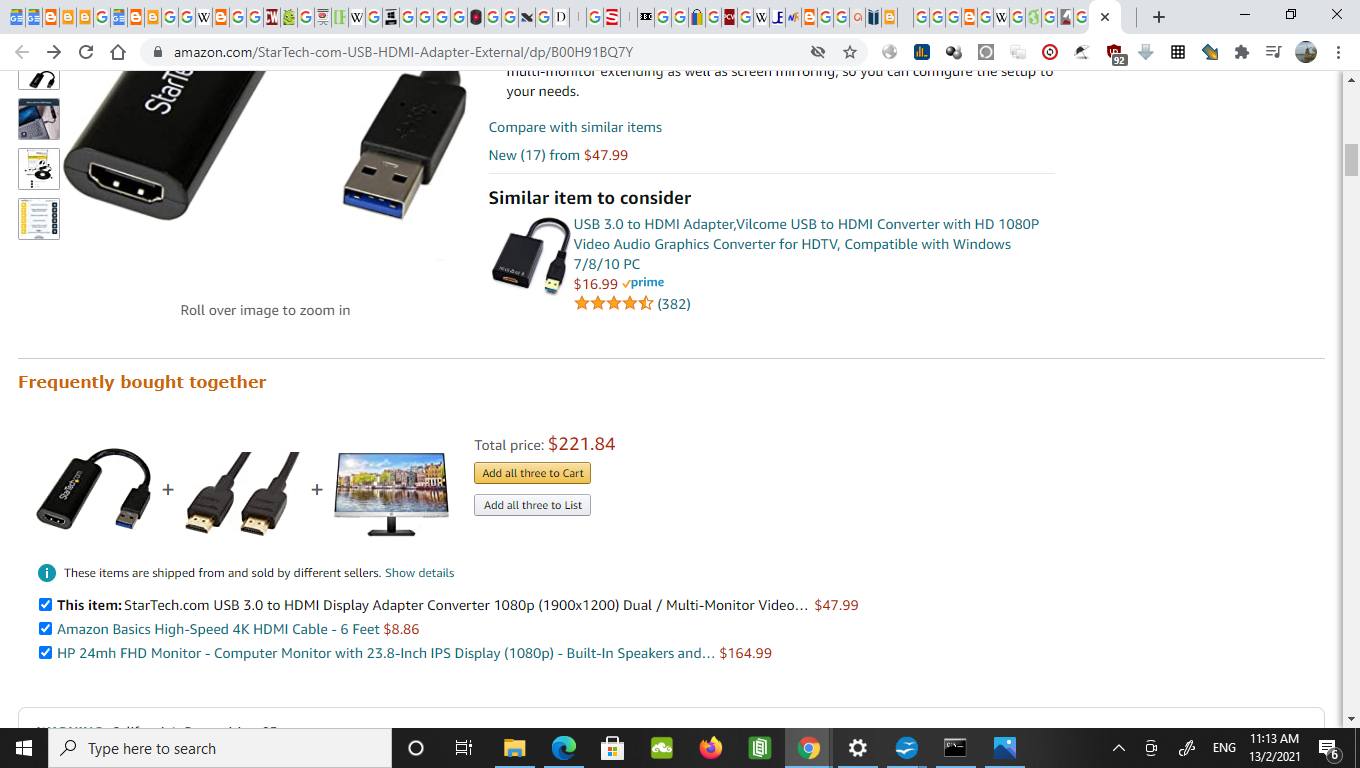This is an advertisement displayed on an Amazon page for a  USB 3.0 to HDMI converter. The converter, priced at $47.99, is designed to connect PCs lacking an HDMI output to HDTVs, offering 1080p HD video and audio compatibility with Windows 7 and 8. The page also suggests related items frequently purchased together, including an Amazon high-speed HDMI cable, HP 24-inch FHD computer monitor, and a USB display adapter converter for multi-video monitoring. The display partially scrolled down, concealing some product details.